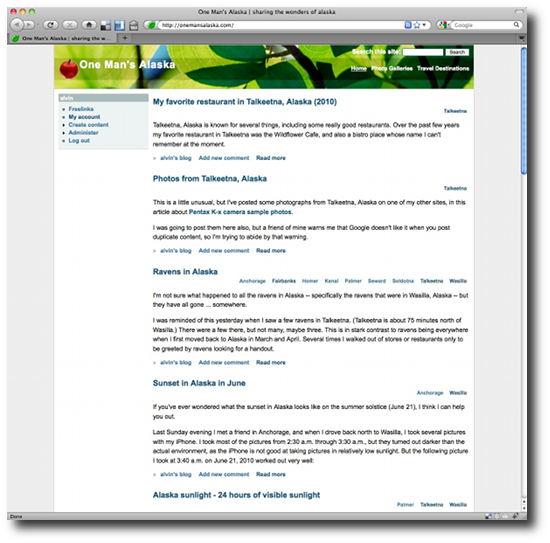Screenshot Description:

This detailed screenshot depicts a web page viewed through an Apple Safari browser. In the upper left corner of the browser window are the typical traffic light buttons: a red, yellow, and green dot. At the top center of the web page, there's a title that reads "One Man's Alaska: Sharing the Wonders of Alaska." In the upper right corner, there appears to be a close button, characteristic of the Apple or Safari interface.

Beneath the title bar, the browser navigation buttons are visible. These include a back button, a forward button, a refresh button, a stop/close button, and a home button. Next to these buttons, there are two square icons, one black and one blue, the purpose of which is unclear.

To the right of these icons is an open envelope symbol, likely for email. Further right is the address bar, which vaguely reads "HTTP..." with an indistinguishable URL, possibly "goingalaska.com." Adjacent to the address bar is an unchecked favorite star icon, suggesting the page is not bookmarked, followed by a drop-down arrow for accessing browsing history.

Further to the right is a Google search bar. Below these navigational elements, the webpage title, "One Man's Alaska: Sharing the..." is partially visible, repeating the main title at the top. The main content area includes a picture of green leaves as a background, with the repeated title "One Man's Alaska" superimposed on it.

To the right of this image, there are several navigation links: "Home," "Photo Gallery," "Travel," and "Destinations."